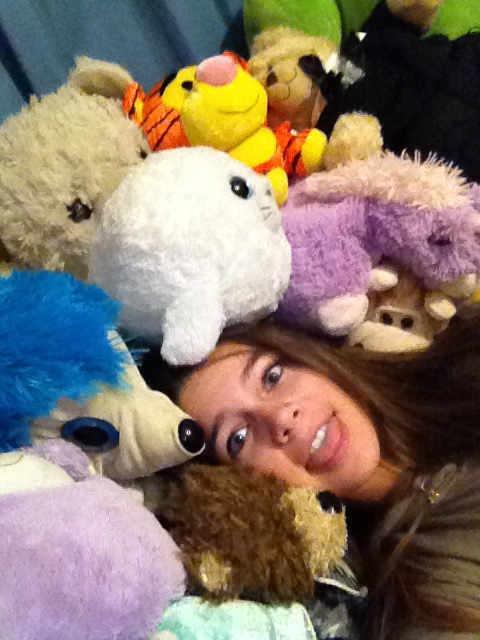In the photograph, a young girl, approximately 12 to 14 years old, lies on her back amidst a sea of colorful stuffed animals with only her head and a bit of her right shoulder visible. She has long brown hair and light skin. Her eyes are wide open, brown, and she gazes directly at the camera with her tongue slightly protruding from her open mouth, revealing a row of straight, white upper teeth. Surrounding her head are various stuffed animals: a variety of brown teddy bears, a distinctive white teddy bear, a character resembling Tigger, a fat white harbor seal, and a white-nosed creature with a tuft of bright blue hair. There are also several purple stuffed animals, one with cream-colored fur on top, a yellow and orange one, and another resembling a blue hedgehog. Additionally, other toys include a dark brown teddy bear, a lighter brown teddy bear, a beige teddy bear with black eyes, a purple horse, and what might be the face of a monkey, as well as some indistinct ones in shades of green and light blue. The plush toys, fuzzy and vibrant, seem to pour around her head, creating a whimsical and cozy scene.